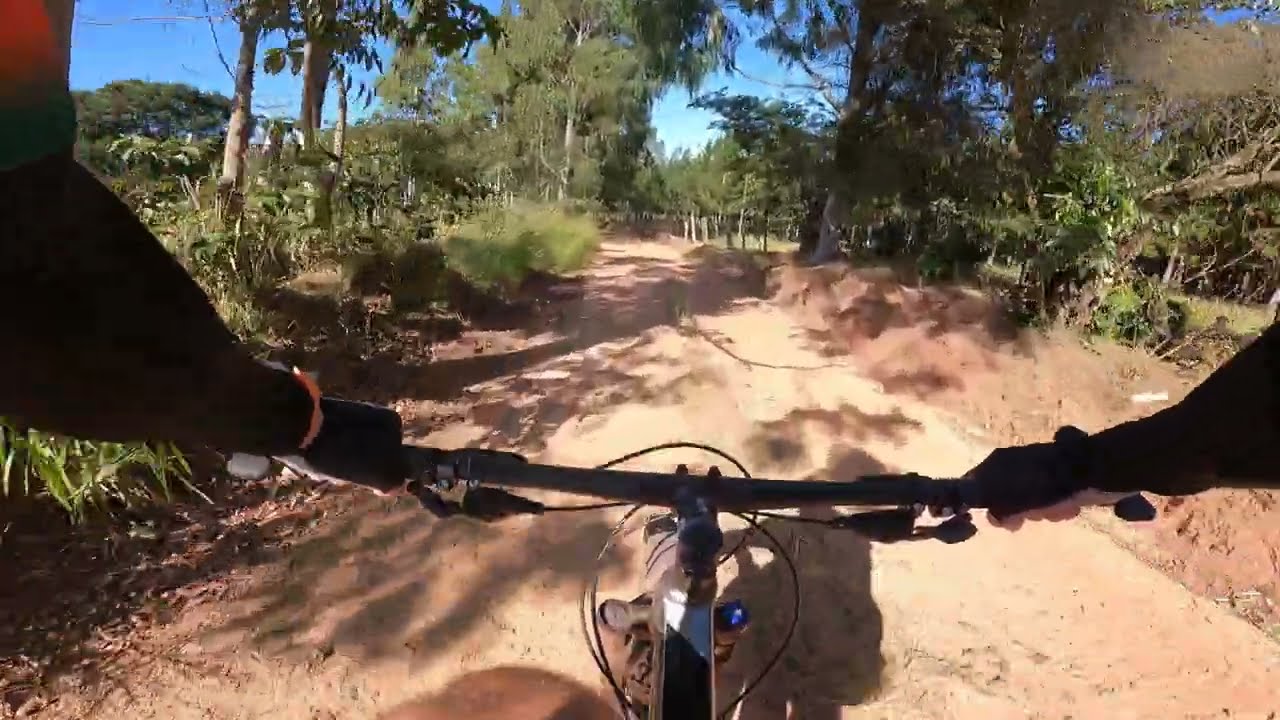A vibrant and sunny day frames the front-facing view of a cyclist navigating a wide dirt path surrounded by lush greenery. The perspective, as if from a camera mounted on the bike's front, captures the cyclist's black-sleeved arms gripping the black handlebars, from which various cables extend. The left wrist features an orange waistband. The dirt path, flanked by green trees, casts intricate shadows across its sandy surface. In the distance, more trees stretch towards a bright blue sky adorned with patches of white clouds. On either side of the path, shrubs and grasses thrive, adding to the rich tapestry of green against the earthy sand. The scene conveys a tranquil outdoor journey, emphasizing the natural beauty and the serene environment.